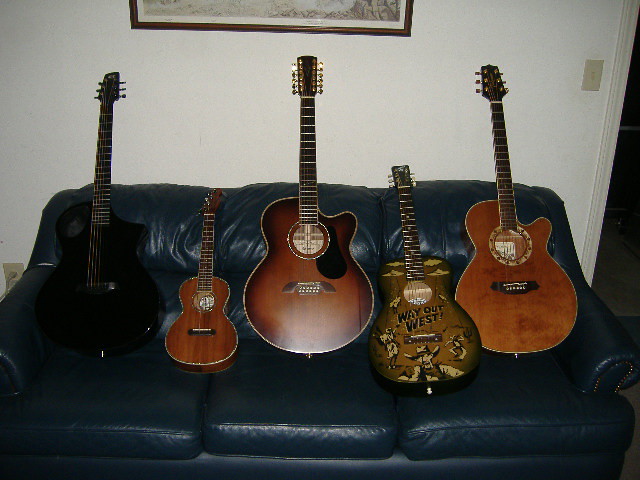The photograph is taken inside a house and shows a black, three-seater couch with arms, positioned against a white wall. A light switch is visible on the upper right-hand edge of the wall, with a doorway partially visible to the right and the bottom edge of a brown picture frame higher up on the wall. On the couch, there are five stringed instruments arranged frets-up. From left to right:

1. A black electric guitar that blends with the couch.
2. A wood-colored instrument, possibly a children's guitar or ukulele, whose top does not extend beyond the back of the couch.
3. A large acoustic guitar, likely a 12-string with a black pick guard.
4. A smaller brown acoustic guitar featuring a "Way Out West" pattern with possible cowboy imagery.
5. Another large, dark brown acoustic guitar.

The majority of these instruments are made from dark wood, adding a rich contrast against the black couch and white wall. The variety in size and design of the guitars adds visual interest, emphasizing a collection of both standard and specialty stringed instruments.